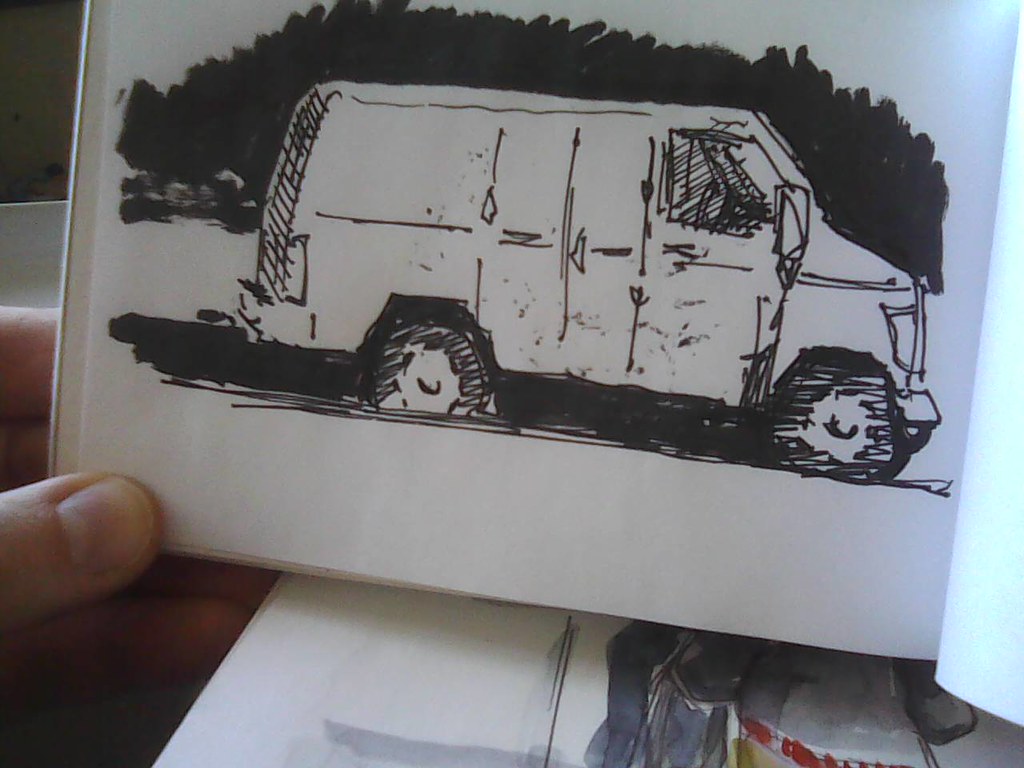The image depicts a hand holding up a piece of paper, likely from a sketchbook, containing a detailed black and white drawing. The drawing, made with black marker or pen, features an old-style, windowless white van, reminiscent of models from the 1970s or 80s. The van is oriented to the right with distinct lines outlining its form and window tint. The background surrounding the van is shaded black, possibly representing trees or a night sky, while the ground beneath the van is also rendered in black to add texture and depth. There is no text in the drawing, and the entire scene is devoid of color, emphasizing its monochromatic aesthetic.